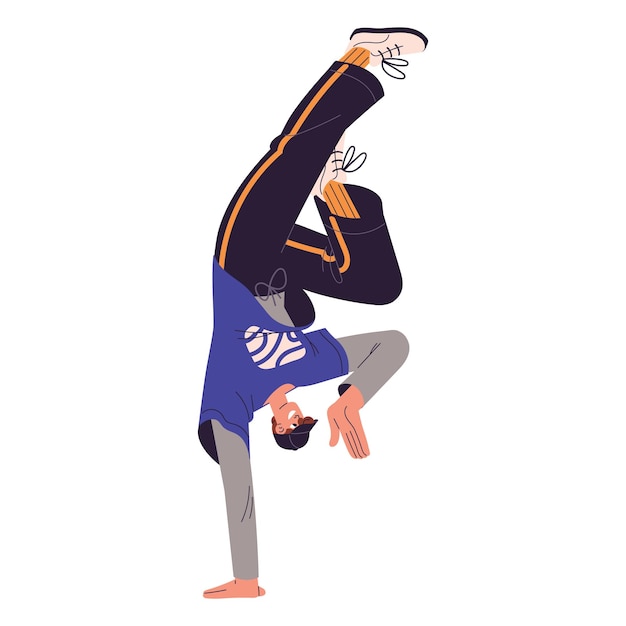The image illustrates a cartoonish Caucasian young man in the midst of performing a one-handed handstand, positioned centrally against an empty white background. He is dressed in an oversized blue t-shirt adorned with a white ball logo, layered over a gray long-sleeve undershirt. His attire is completed by a pair of dark sweatpants featuring orange or white stripes on both sides, yellow socks with black stripes, and white sneakers that have black soles and laces. The man, who has orange hair and wears a black baseball cap, appears to have a small head in proportion to his body and exaggerated large hands. His left hand supports his upside-down stance, while his right hand is bent and positioned near his head. His body is slightly contorted to the right, with his right leg curled and angled, and his left leg extended straight up. He is smiling, exuding a sense of happiness and satisfaction in his athletic pose.